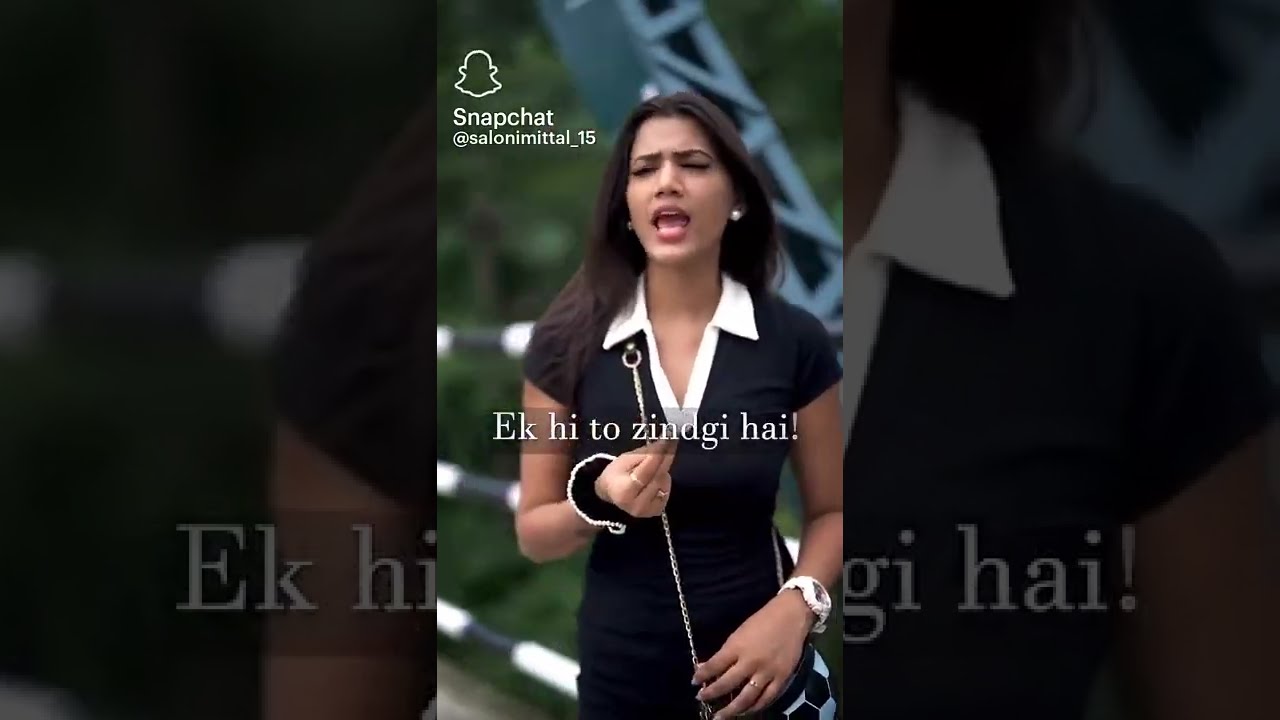In this image, we have a screenshot of a Snapchat post by the user @salonimittal_15. The top-left corner features the Snapchat logo. The post includes text in a foreign language, written as "E-K H-I T-O T-O Z-I-N-D-G-I H-A-I!" The central figure is a young woman, likely in her early 20s, who appears to be talking or singing. She is dressed in a short-sleeved black dress with a white collar and a deep V-neck bordered in white. She accessorizes with pearl earrings, a watch with a white band on her left wrist, and a black and white hair tie on her right wrist. Additionally, she has rings on her right fingers. Her chest-length hair falls around her shoulders. A small purse, featuring a chain strap, crosses her body. In the background, nearly obscured, are some green trees, indicating an outdoor setting. The image captures her mid-action, adding a dynamic element to the scene.